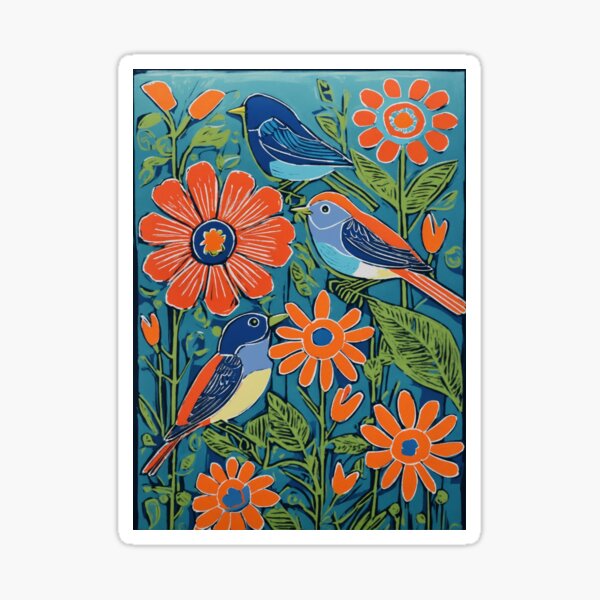This beautifully detailed folk art painting showcases three vibrant birds perched on a cluster of flowers. The top bird features a striking dark blue plumage with lighter blue on its belly and hints of blue in its wings, facing slightly away from the viewer. The middle bird, adorned in three shades of blue—dark, medium, and teal—displays a red head, white accents, and a red tail. The bottom bird mirrors the middle one with a blue head, patches of red down its back, and a yellowish belly. Its feathers are a mix of dark and medium blue with a bold orange tail. Surrounding the birds are vividly colored red and orange daisy-like flowers with blue centers, set against a backdrop of green leaves. The background is a stunning gradient, blending dusky blue into a pale teal, seamlessly integrating all the colors and elements into a cohesive and captivating scene.